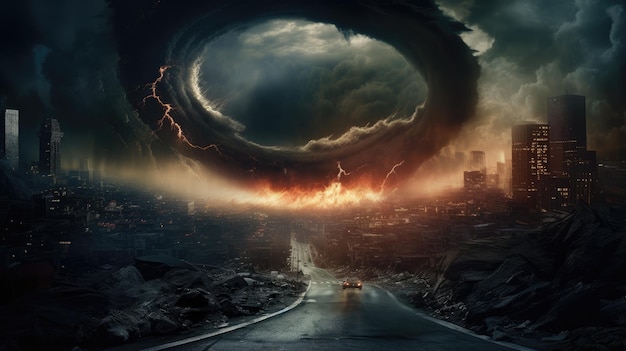A scene of desolation and chaos unfolds in this dark, apocalyptic image. A solitary car, its headlights piercing the gloom, drives along a wet, blackened roadway that winds through utter devastation. To the sides of the road, heaps of crumpled debris hint at once-standing structures now fallen into ruin. Toward the horizon, the dim outlines of high-rise buildings emerge from a backdrop shrouded in ominous, swirling gray smoke. Above, a vast, circular cloud formation—resembling the eye of a storm or the onset of a tornado—hangs menacingly in the sky. This cloud mass is punctuated by sporadic, lightning-like sparkles, adding a surreal sense of foreboding. Below this smoky halo, fiery hues paint the lower sky, intensifying the scene’s apocalyptic feel. Dark clouds loom, with the overall atmosphere suggesting the aftermath of a catastrophic event, evoking a sense of doom reminiscent of a disaster movie. The eerie mismatched illumination, possibly from a setting sun or ethereal flames, casts an otherworldly glow on the landscape, amplifying the scene’s unsettling, end-of-times ambiance.